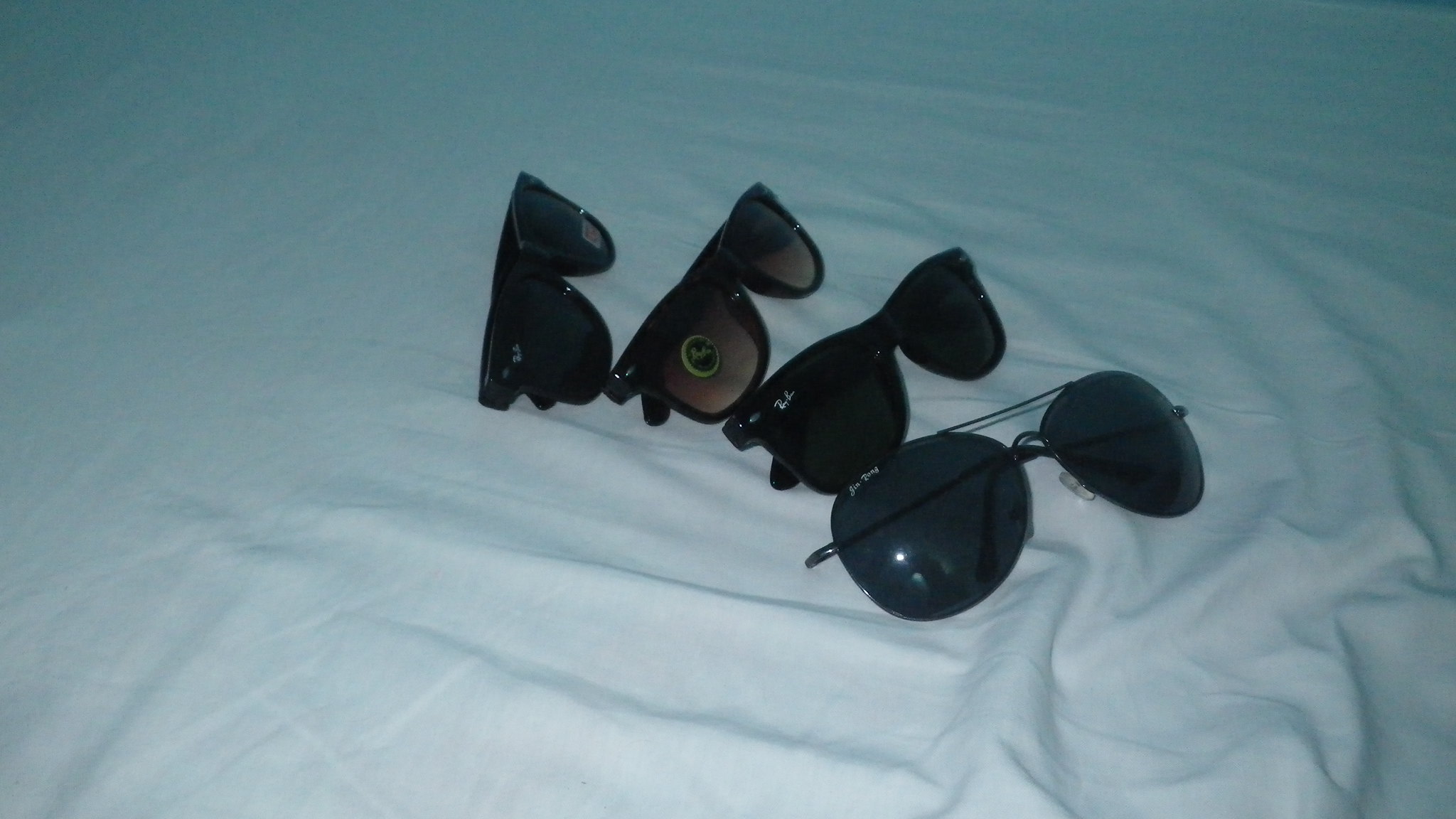A photograph features four pairs of sunglasses, all arranged in an arch on a wrinkled white sheet. The first pair, positioned at the top, features black plastic frames with dark lenses, and a small label on the left lens. The second pair has black plastic frames with amber-colored lenses that transition to gray, and a sticker on the right lens. The third pair, resembling the first, also has black plastic frames and dark lenses, marked with the Ray-Ban logo on the right side. The fourth pair, situated on the bottom, is an aviator style with thin metal rims connecting the larger rounded lenses, also branded with Ray-Ban. The arrangement varies from vertical at the top to almost horizontal at the bottom, the sheet beneath them slightly gathered on one side.